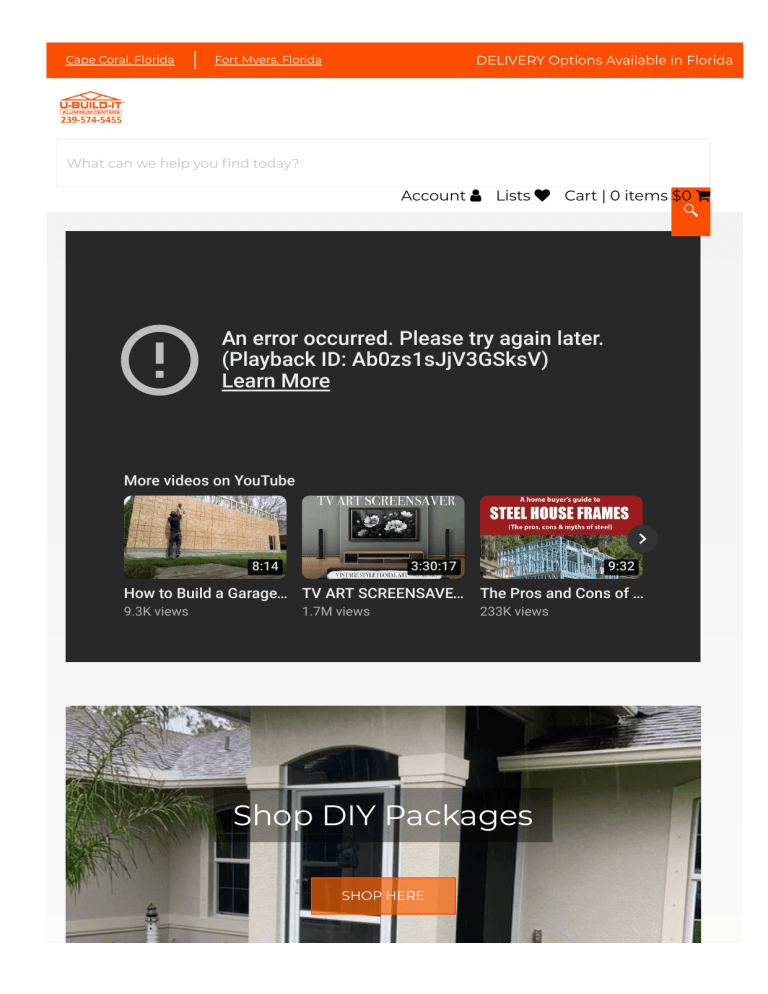**Detailed Caption:**

The webpage features an orange header boldly stating "Delivery options available in Florida." At the top right, various utility icons are neatly aligned: a profile icon, a wishlist represented by a list with a heart, and a shopping cart showing zero items and a total of zero dollars. Below the header sits a white search bar accompanied by an orange square icon to initiate the search.

A notification circle with an exclamation mark alerts users about an error message saying, "An error occurred, please try again later (playback ID: letters and numbers)." This is followed by links to "Learn more" and "More videos on YouTube."

The page includes a series of video thumbnails with overlay text. The first video, titled "How to build a garage..." has a duration of 8 minutes and 14 seconds. Another video spans 3 hours, 30 minutes, and 17 seconds and is titled "TV art screen save...". Below it is a 9-minute and 32-second video titled "The pros and cons of...".

At the bottom of the page, an image of a house is displayed above a gray rectangular banner adorned with the words "Shop DIY packages." Adjacent to this, an orange rectangle stands out with the call-to-action text "Shop here" written in white.